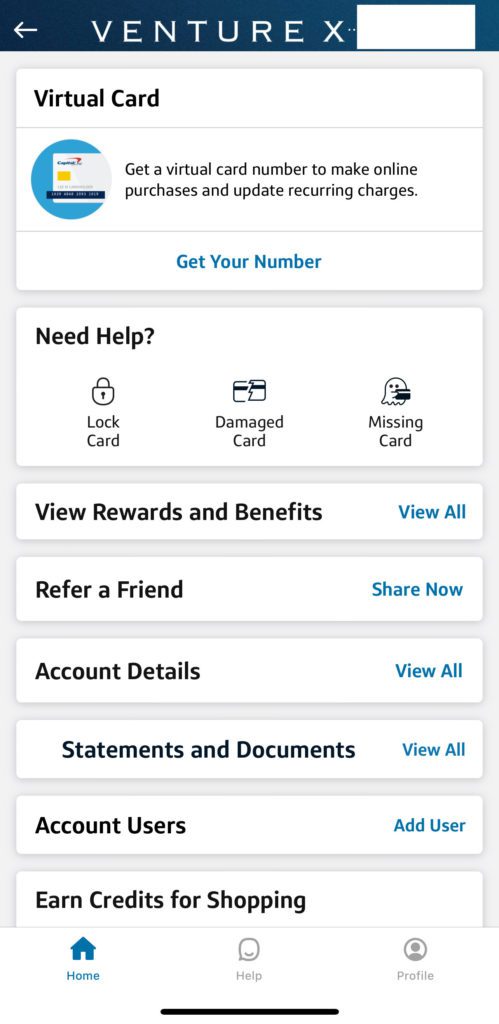Here is a more concise and detailed caption for the described screenshot:

---

The screenshot depicts a financial app named "Venture X" on a smartphone. At the top, a section titled "Virtual Card" offers users the ability to obtain a virtual card number for online purchases and recurring charges, accompanied by a cartoony credit card icon. An option to "Get Your Number" is available in blue text for initiating the process.

Below, the "Need Help" section features various support options: "Lock Card," "Damaged Card," and "Missing Card," each with respective icons illustrating a lock, damaged card, and ghost holding a card.

Further down, several more sections provide accessible features:
- "View Rewards and Benefits" with a "View All" link
- "Refer a Friend" with a "Share Now" option
- "Account Details" with a "View All" link
- "Statements and Documents" with a "View All" link
- "Account Users" with an "Add User" link
- "Earn Credits for Shopping," partially visible

The bottom navigational bar of the app includes icons and labels for "Home," "Help," and "Profile," indicating primary navigation options for the user.

---